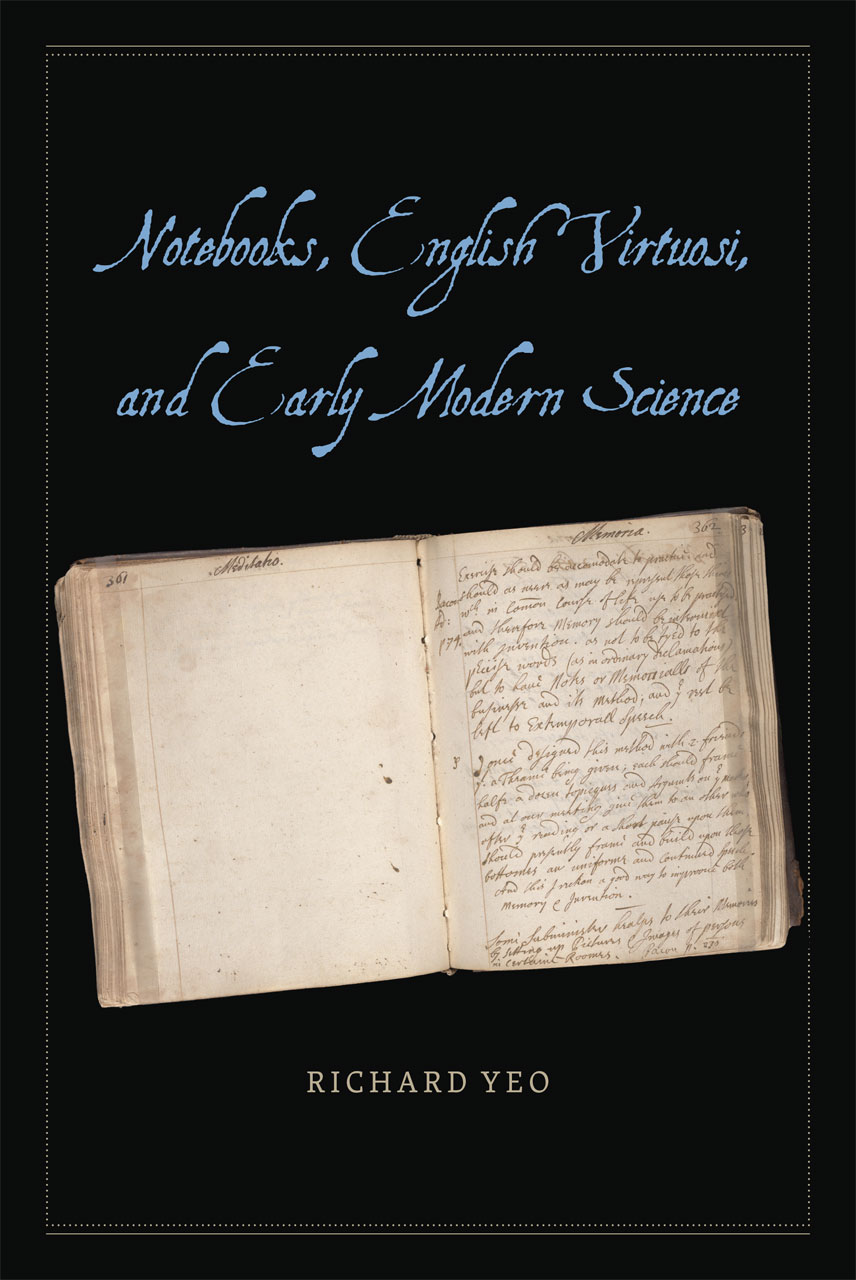The poster features a solid black background framed with a border of white dots. At the top, in elegant blue cursive lettering, the text reads: "Notebooks, English Virtuoso, and Early Modern Science." Below this, at the center, is an image of an open notebook with an aged parchment appearance, displaying a blank left page and a right page filled with small cursive writing in pale black ink. The notebook pages are a cream to light beige color, complementing the ink. Beneath the notebook image, the name "Richard Yeo" is prominently displayed, indicating the author or presenter. The overall design evokes a scholarly and historical aesthetic, reminiscent of early modern scientific manuscripts.